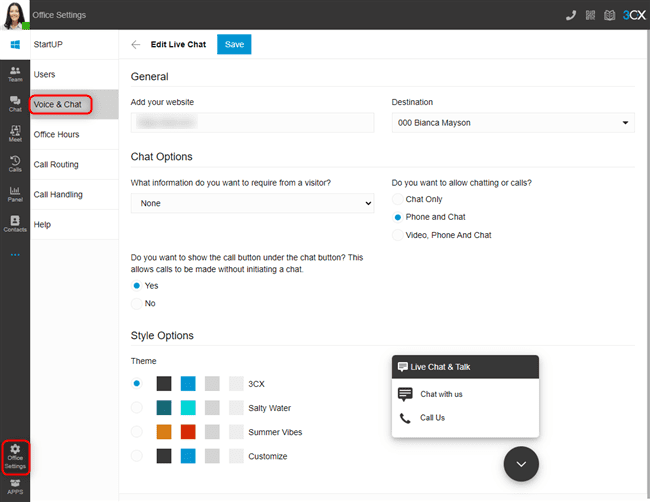The image depicts a detailed chat options settings page with a white background and black rectangular headers at the top and along the left side. In the upper left corner, there is a photograph of a smiling Caucasian female with shoulder-length brown hair and light skin. To the right of her image, white text on the black background reads "Office Settings." Further to the right, there are a phone icon, two other small icons, and the text "3CX."

Below this header, on the left, are several key elements displayed in a systematic layout:
- A Windows icon, followed by black text that reads "Startup," next to a left-pointing arrow and the text "Edit Live Chat."
- To the right of these icons is a blue rectangular button with white text that says "Save."
- A section labeled "Users" followed by "General," both in black text.
- Below this, a gray rectangular section containing another red-outlined rectangle. Inside this section, the black text reads "Voice and Chat" followed by "Add your website," with the website portion blurred out.
- Text labeled "Destination," followed by "000BiancaMason" next to a dropdown menu.
- Sections for "Office Hours," "Call Routing," and "Call Options."
- Another section labeled "Call Handling," followed by the query, "What information do you want to require from a visitor?" with a dropdown menu set to "None."
- Options below this query include: "Do you want to allow chatting or calls?" with choices "Chat only," "Phone and Chat," and "Video, Phone, and Chat."
- Further down, a "Help" section.
- An inquiry that says, "Do you want to show the call button under the chat button? This allows calls to be made without initiating a chat," followed by options "Yes" and "No."
- Finally, a section for "Style Options."

At the bottom right of the page, there are options labeled "Live Chat and Talk," "Chat with Us," and "Call Us."